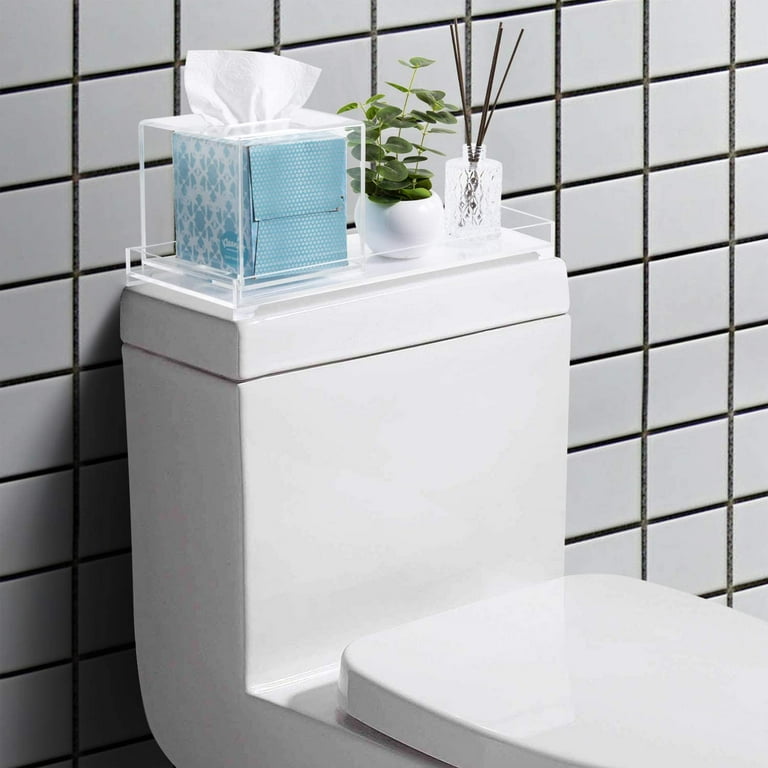This is a detailed, zoomed-in photograph of a modern bathroom focusing on a standard white toilet. The walls are tiled with crisp, clean white tiles that feature thin, black lines running both horizontally and vertically, creating a grid pattern. The toilet itself has a rectangular, square tank with an oval lid. On top of the tank, there is a clear glass box containing a blue tissue box, a small, green shrubbery plant in a white flower pot, and a transparent oil diffuser with brown sticks. The photo is sharply focused and does not contain any text.